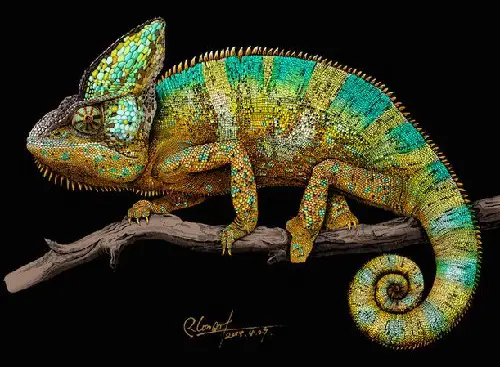In this digital artwork, a chameleon with a striking mix of colors and textures perches on a slender, brown tree branch against a pitch-black background. The chameleon, positioned facing left, boasts a yellow ear and a vibrant combination of green, yellow, and blue along the top of its face and back. Detailed line segments enhance its back, while numerous tiny spikes adorn the top of its head and along its jaws. Its four legs grasp the branch tightly, and the chameleon's tail curls elegantly to the right beneath the branch. The detailed textures give the impression that the chameleon might be crafted from beads, adding a unique, tactile quality to the artwork. A signature, located at the bottom center of the image, suggests it could be a piece created to showcase the artist's skill.